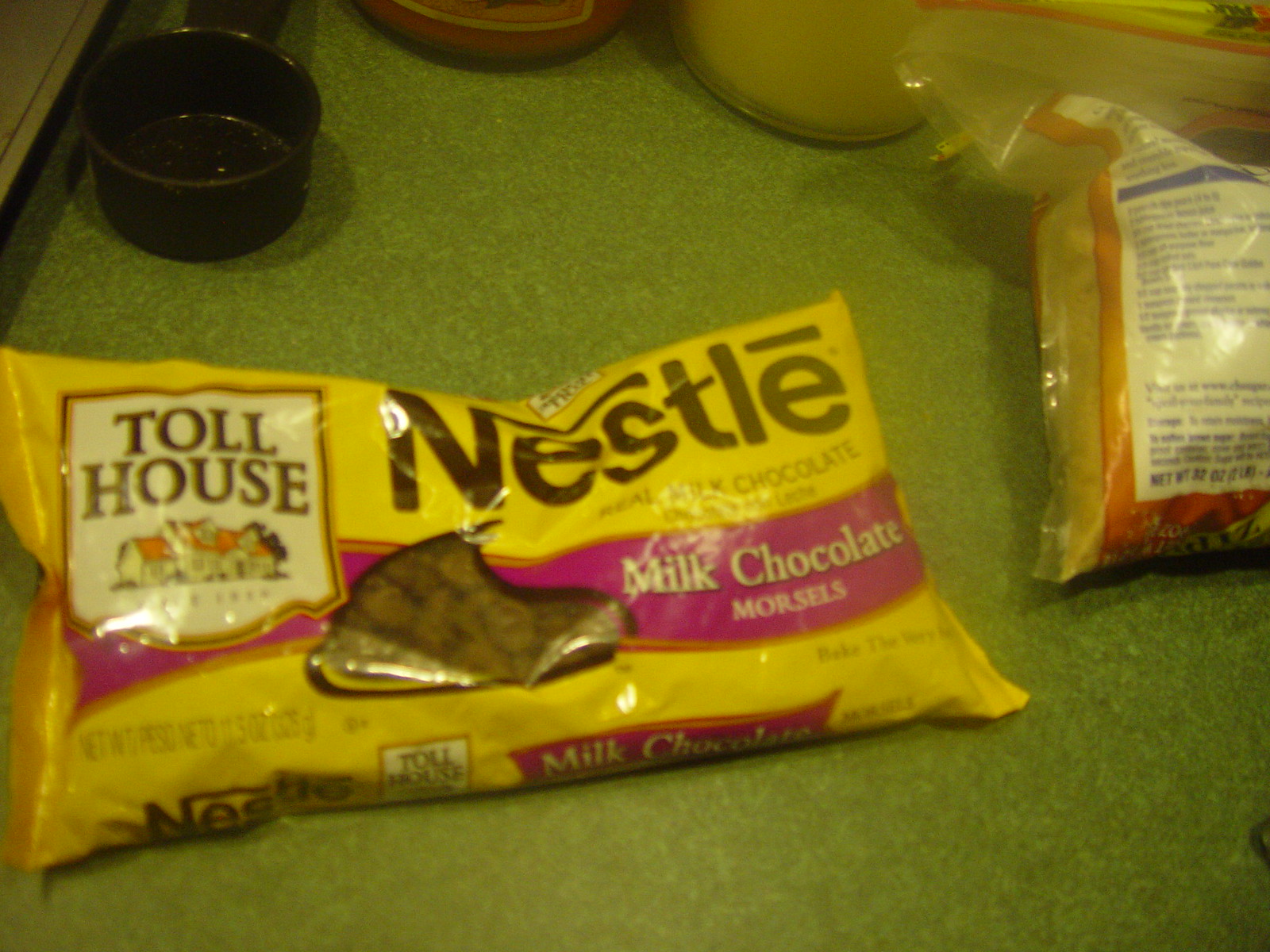This detailed photograph captures a lively kitchen scene centered around baking preparations. Dominating the green counter is a brightly colored bag of Nestle Toll House milk chocolate morsels, easily identifiable by its yellow and pink packaging. Beside it lies an inverted bag of brown sugar, displaying its ingredients and possibly a recipe on the back. A solid black measuring cup is positioned just behind the bag of chocolate chips. Partially visible at the edge of the frame are the bottoms of two jars, adding to the sense of a bustling kitchen in mid-preparation. Adjacent to the counter, a raised surface hints at further kitchen activities beyond the frame.